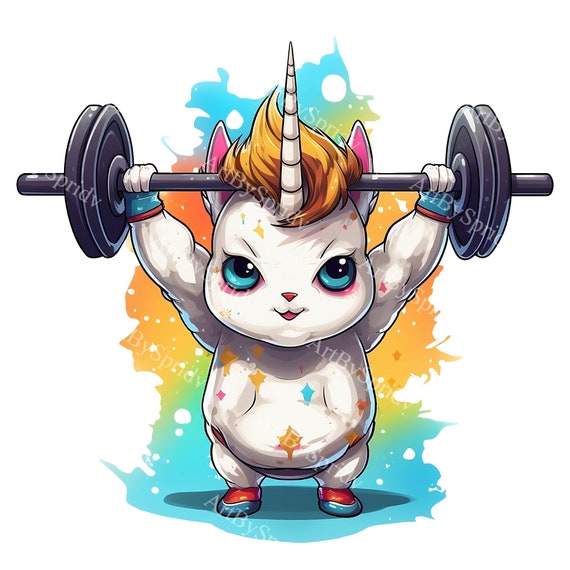This digital cartoon illustration features a chubby, muscular unicorn character standing on its hind legs, holding a barbell above its head in a determined pose, as if in the midst of an intense workout. The unicorn has blue eyes, a blondish mane, and pink ears, clearly indicated by the characteristic horn protruding from its forehead. Its stocky, stout form resembles a blend of human and animal features, complemented by muscular arms and a round belly. Adorning red and blue shoes, the unicorn adds a touch of whimsy to its otherwise robust appearance. The background of the image is a white square with splashes of vibrant colors including blue, yellow, and orange, reminiscent of paint splatters, which highlights the energetic and spirited essence of the scene.